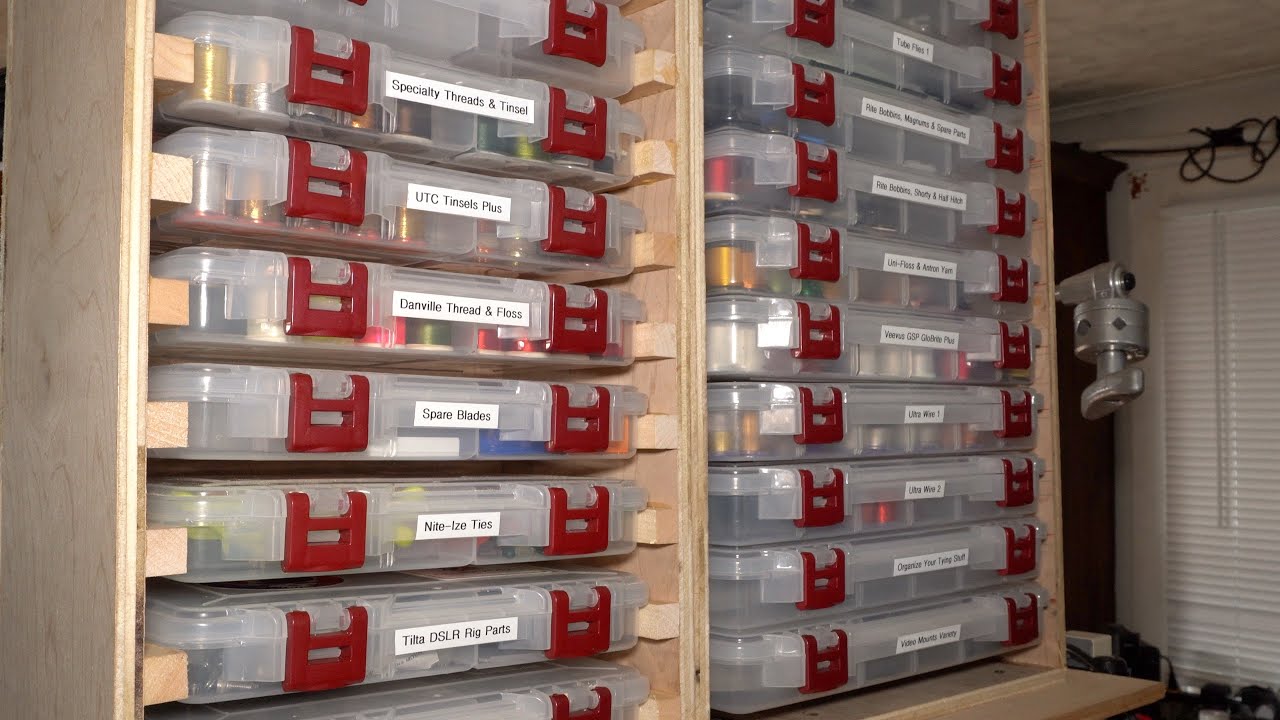The image depicts a room with a large wooden shelving unit at its center, meticulously organized with clear plastic containers that have red latches. Each container is labeled with a white tag featuring black text. Visible labels include "Specialty Threads and Tinsel," "UTC Pencils Plus," "Danville Thread and Floss," "Spare Blades," "Night Ties," and "Tida DSLR Rig Parts." The shelving unit has square compartments that perfectly accommodate these containers. To the right, another room is partially visible, featuring white horizontal blinds and a metallic contraption that resembles a tool, possibly something like a sander, suggesting a workshop or garage setting. A hint of a black curtain hangs near the window, but it is partially obscured by the shelving unit. The organized setting and specific labels suggest a space dedicated to crafts or tools, adding to the sense of meticulous order and functionality.